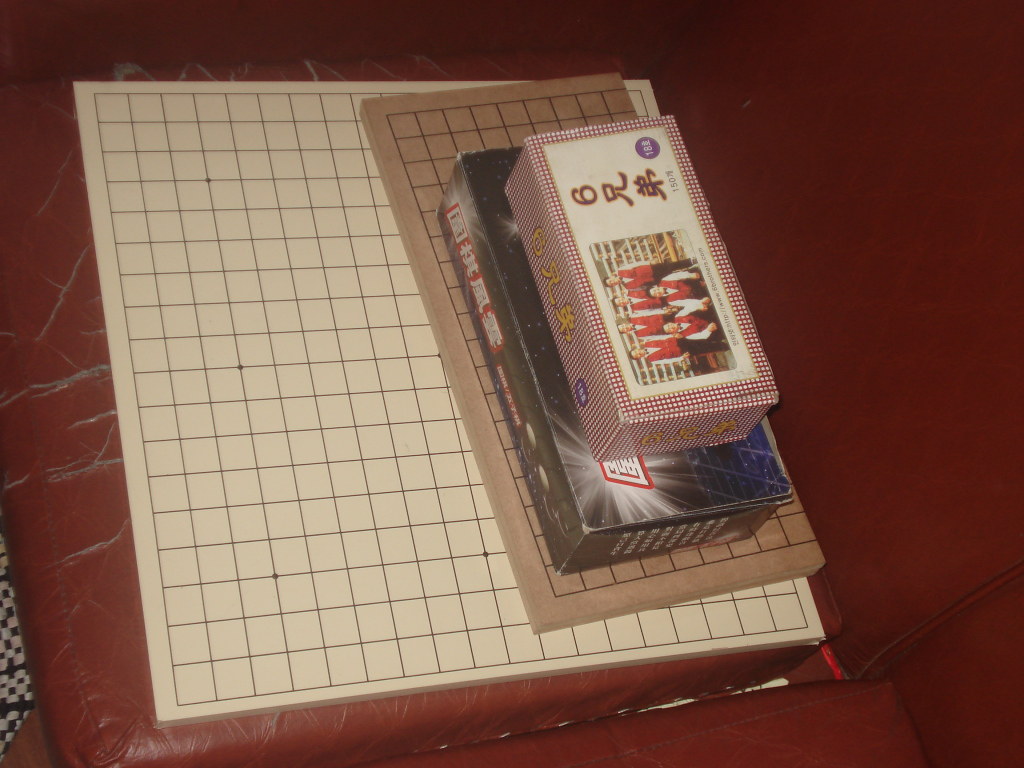This is a highly detailed color photograph depicting a stack of various objects arranged on a worn, reddish-brown leather couch cushion. The cushion shows signs of wear and tear, with visible discoloration and cracks in the leather.

At the base of the stack is a leather-like item, possibly a folder or notebook. Directly on top of this lies a large, whitish-beige board covered with a grid pattern resembling graph paper, marked with black squares. This board occupies a substantial portion of the visible area.

Perched on this large board is a smaller, brown game board that also features a pattern of squares outlined in black. This smaller board covers approximately half of the larger board’s surface.

Above these boards, two rectangular boxes are stacked. The lower box is darker in color and features Asian writing, possibly Japanese or Chinese, along the spine. The top-most box is more colorful, with a white center showcasing an image of several people dressed in red vests and dark pants. The design elements on this box are predominantly red, white, and black, contributing to an abstract aesthetic.

The entire stack is set against a backdrop that might be maroon, suggesting it could be the color of the table or additional background elements.